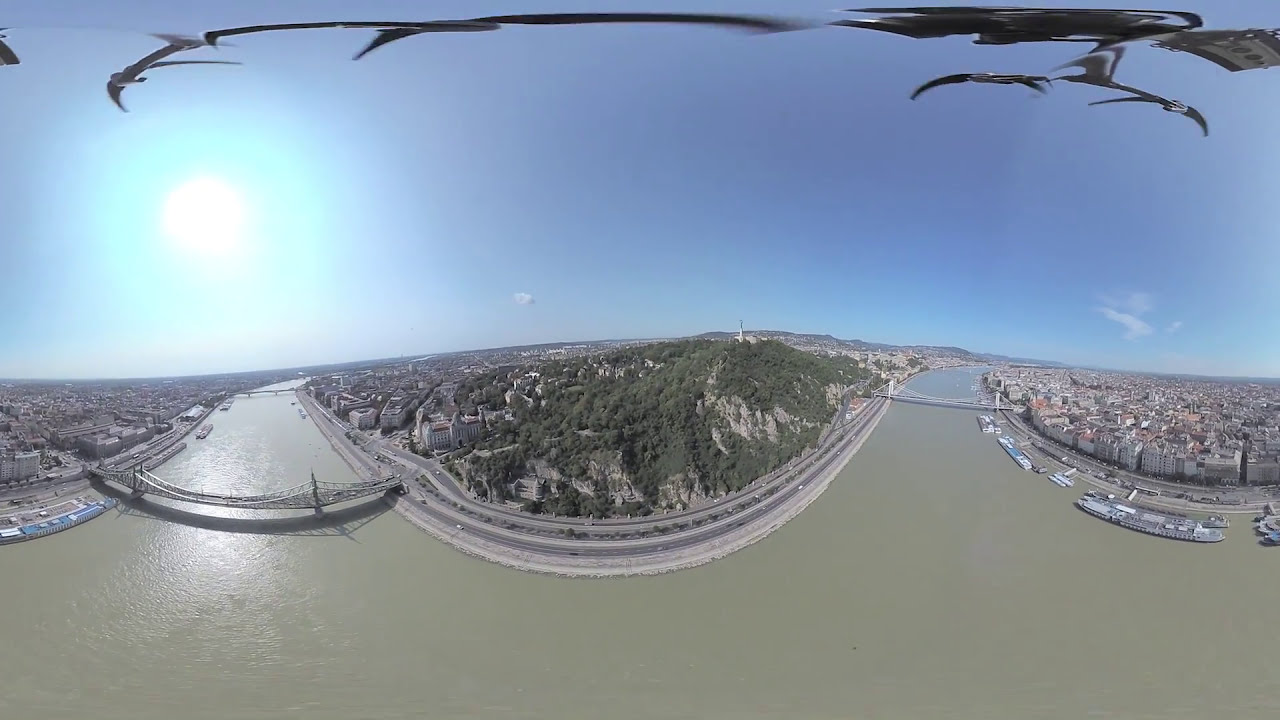This panoramic shot, taken from a drone, captures a scenic river landscape. The river, while appearing to curve due to the panoramic nature of the photograph, likely flows straight in reality. The water initially appears olive-colored and muddy but turns a striking blue past a bridge on the right side. The sky above is a clear, vibrant blue with the sun positioned in the upper left corner, producing a glare of lighter yellow and green hues. The drone's black ends and possible distortions, appearing as thin and straggly black strips, are visible at the top of the image.

In the center of the photograph lies an old European town with a mix of small buildings and trees. This town extends predominantly towards the right side of the image. On the left, a bridge emerges from a mountainous area, connecting this natural landscape to the town's outskirts. Another bridge on the right crosses into a more developed region characterized by apartment buildings, larger docks, and further residential homes.

Overall, the image captures a harmonious blend of nature and human habitation, with the serene blue skies and contrasting river waters setting a picturesque background for this quaint European town split by the bridging river.